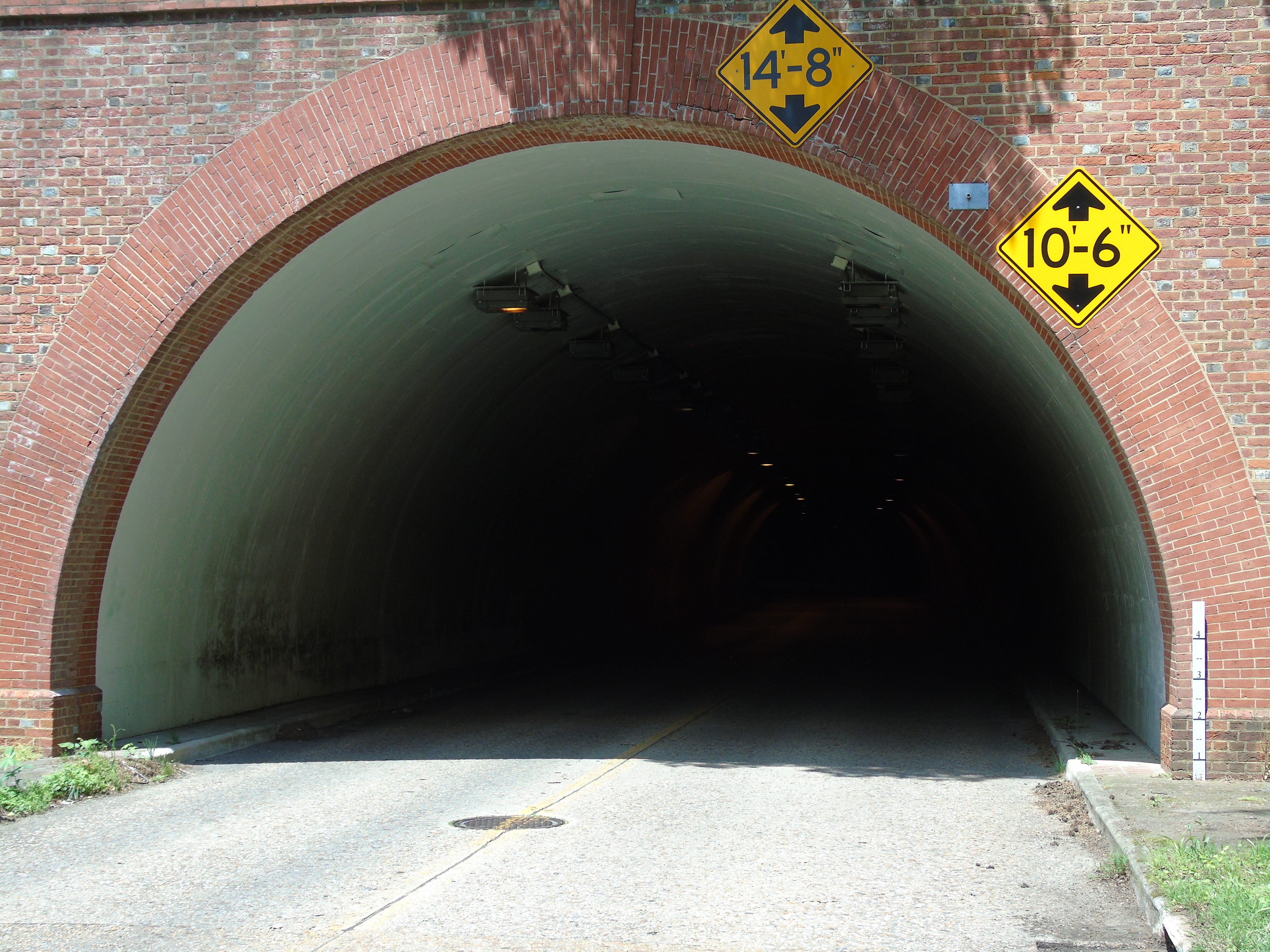The photograph captures the entrance to a road tunnel constructed with red and gray bricks. The archway of the tunnel prominently displays two height restriction signs: one at the very top indicating "14 ft 8 in," and another on the right-hand side, closer to the ground, displaying "10 ft 6 in." These signs, featuring yellow backgrounds with black arrows, warn drivers regarding vehicle height. The road leading into the tunnel is a two-lane passage marked by yellow center lines and includes a manhole cover. The tunnel itself quickly descends into darkness, with the interior appearing pitch black except for faint overhead lights that do not fully illuminate the passage. The curvature of the tunnel showcases a white-painted ceiling, contrasting the brickwork of the entrance and providing a glimpse of the tunnel's rounded structure.